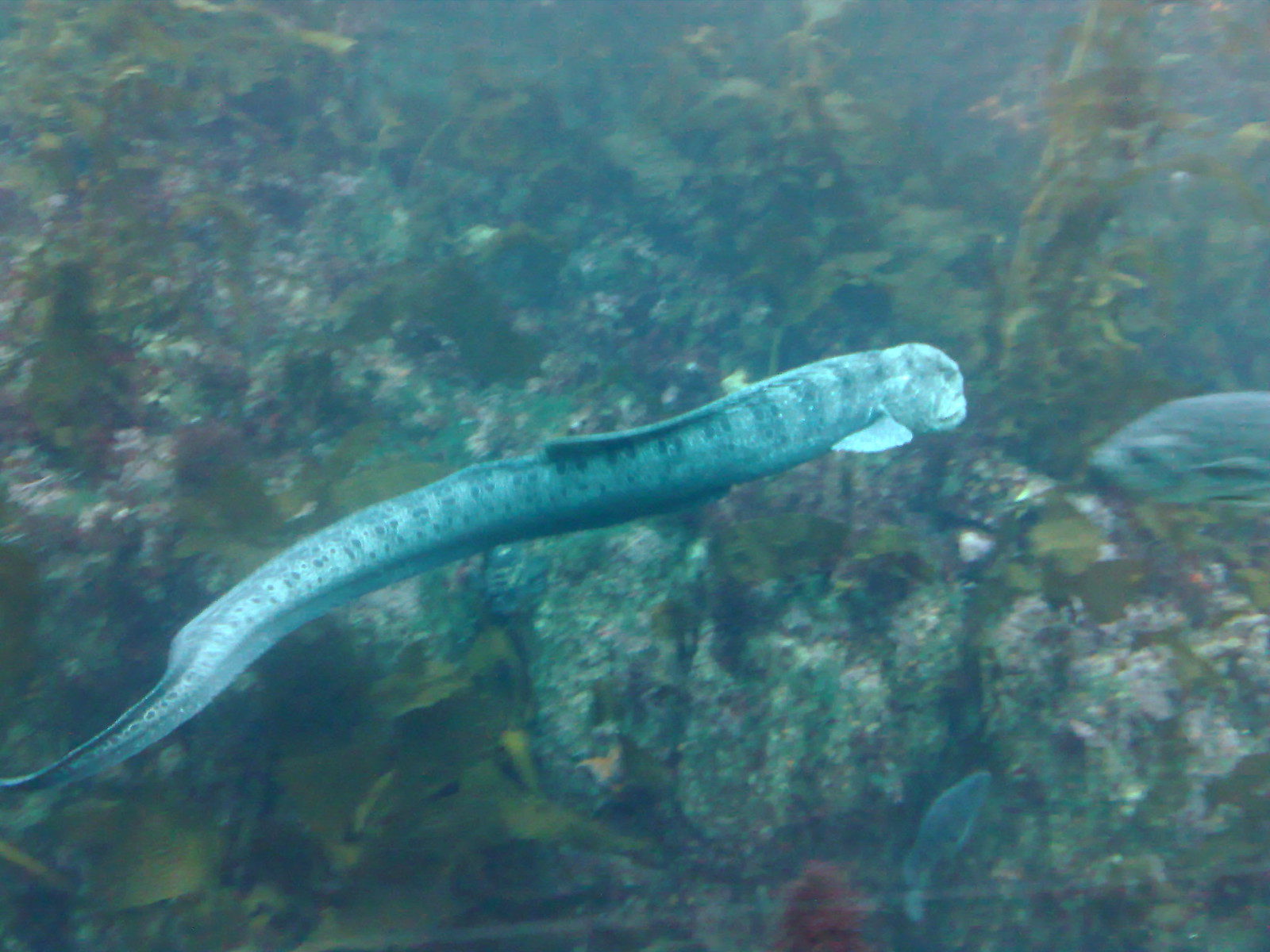The underwater image depicts a dynamic and vibrant marine scene featuring a prominently long, slender sea creature, most likely an eel, with distinct black and blue striped patterns along its elongated, cylindrical body. The eel has a square-ish head with a small fin just below, and a tail that tapers to a thin point, adorned with subtle white circles. The eel appears to be swimming gracefully without noticeable fins, creating a slithery effect.

Surrounding the eel, the ocean floor is teeming with life. It's densely covered with green leaves and moss, suggesting a thriving underwater ecosystem. The rocky background further enhances the image's depth, with rocks appearing white and gray, textured with patches of green, yellow, and brown moss.

Additional details include various small fish darting around the scene: a blue fish with a green bottom belly swimming in from the right, and another blue fish with a yellow or green belly seen swimming upward from the bottom. Blurry movement from the left hints at more fish activities. The tank water itself has a dark blue-green hue. A hint of red, possibly from a plant growing in the lower right corner, adds a pop of color to the vivid underwater landscape.